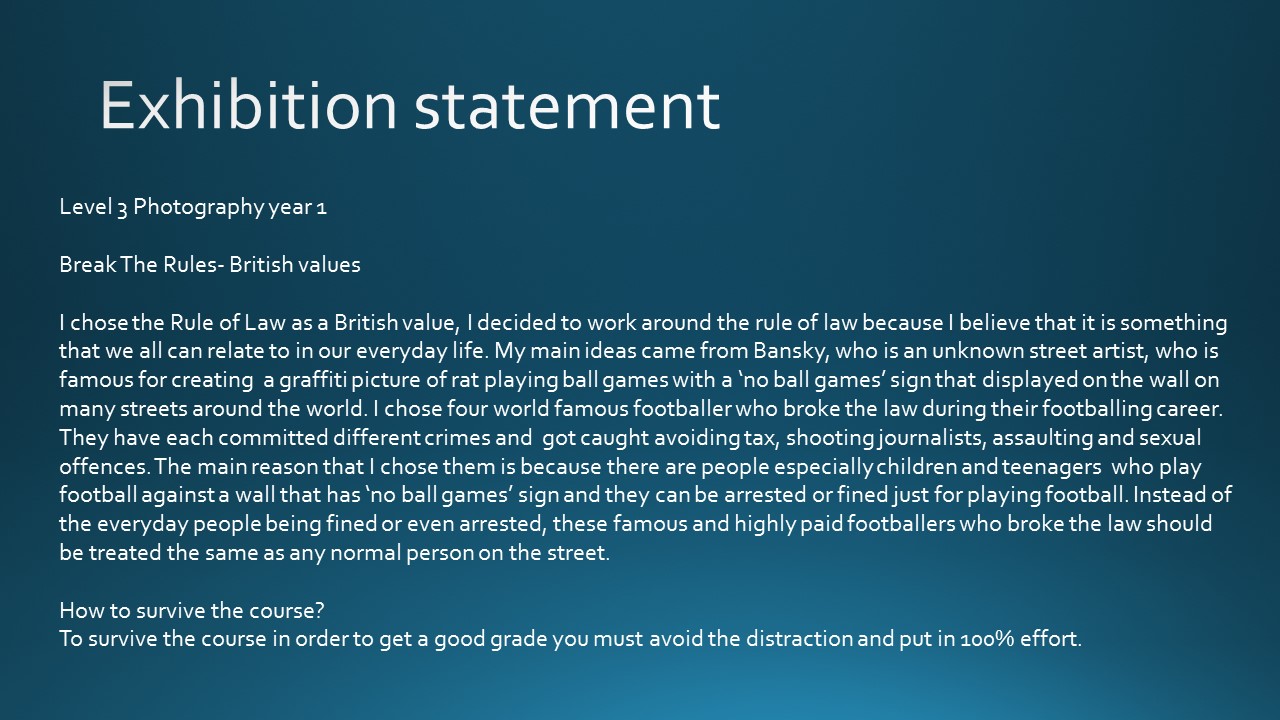The image features an exhibition statement on a turquoise background that transitions to a lighter shade towards the bottom and darkens at the sides and top. At the top of the image, in large white letters, it says "Exhibition Statement." Directly below this, in smaller white text and a different font, it reads, "Level 3 Photography Year 1," followed by "Break the Rules - British Values."

The main body of text starts with the declaration, "I chose the rule of law as a British value." The author explains their focus on the rule of law, stating that it is a concept we all can relate to in our everyday lives. The text further elaborates that the primary inspiration for the project comes from Banksy, a famous but anonymous street artist known for his graffiti artworks. One example mentioned is Banksy's creation of a graffiti picture featuring a rat playing ballgames next to a "no ballgames" sign displayed on walls in multiple locations globally.

The statement continues with a personal reflection on how to succeed in the photography course, titled "How to Survive the Course." It advises that to achieve a good grade, one must avoid distractions and put in 100% effort.